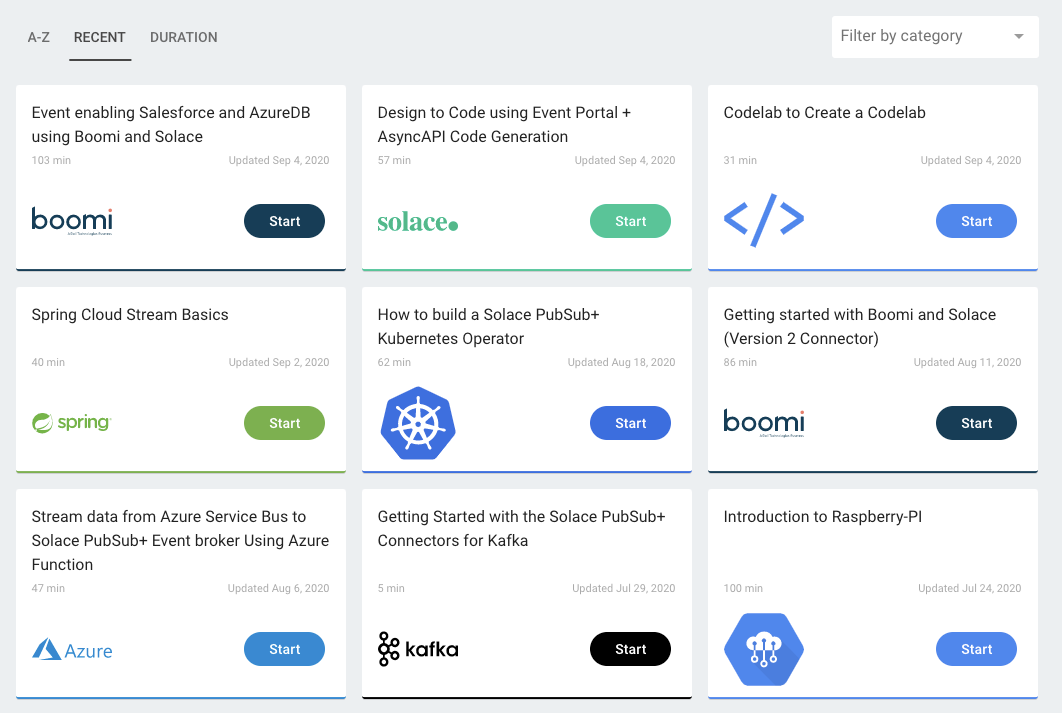The page displays various options organized in a 3x3 grid layout of thumbnail-sized rectangles. Each thumbnail represents an activity or tutorial related to various technologies. The thumbnails can be sorted by "A to Z," "Recent," or "Duration," with the "Recent" option currently underlined. A filter option is located on the far right allowing users to filter by category.

### First Row (Left to Right):
1. **Boomi**: "Event enabling Salesforce and Azure DB using Boomi and Solace." A blue "Start" button is available.
2. **Solace**: "Designed to code using Event Portal and Async API code generation." Features a light blue "Start" button.
3. **Code Lab**: "Create a Code Lab." Includes a symbol of two arrows with a slash through them and a different shade of blue "Start" button.

### Second Row (Left to Right):
1. **Spring Cloud Stream Basics**: Comes with a green "Start" button.
2. **Solace Pub Sub Plus**: "How to build a Solace Pub Sub Plus Cooper meets Operator." Includes a blue "Start" button.
3. **Boomi & Solace V2 Connector**: "Getting started with Boomi and Solace version 2 connector." A blue "Start" button is available.

### Third Row (Left to Right):
1. **Azure Function**: "Stream data from Azure Service Bus to Solace Pub Sub and Event Broker using Azure Function." Comes with a blue "Start" button.
2. **Solace Connectors for Kafka**: "Getting started with the Solace Pub Sub Plus Connectors for Kafka." Displays the company logo and a black "Start" button.
3. **Raspberry Pi**: "Introduction to Raspberry Pi." Features an icon of a blue hexagon with a white cloud in the middle and a blue "Start" button.

This organized layout and detailed labels make it easy to navigate and identify various tutorials and activities available on the webpage.